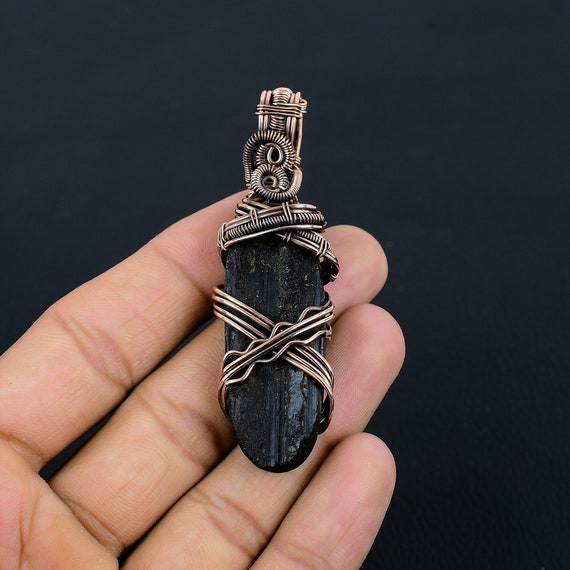The image portrays a left hand emerging from the bottom left corner against an entirely black background. The hand displays four fingers, notably absent of the thumb, and delicately supports a black, rounded stone. This stone exudes a sophisticated, polished appearance, although it is imperfect with faint scratch markings. It is intricately wrapped in a coiled, brassy metal design that forms an 'X' across its center. Additionally, decorative metal strands partially spiral around the stone, enhancing its pendant-like quality. These metal coils, adorned with springs and a clip at the top, suggest that the object is designed to be worn as a part of a necklace. The detailed craftsmanship of the metalwork stands out against the stark black background, emphasizing the stone's elegant and ornamental purpose.